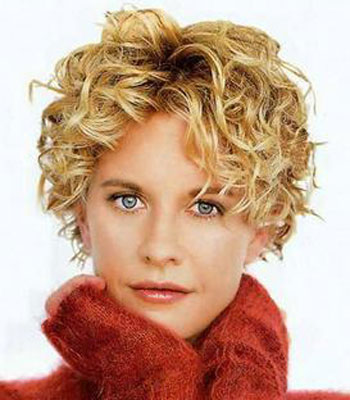This image features Meg Ryan against a completely white background, centered within the frame. Meg Ryan's short, tousled, blonde hair with darker roots frames her face as she looks directly at the camera with a neutral, slightly interested expression. Her striking blue eyes and light peachy lipstick add a touch of color to her face. She is dressed in a cozy, furry, burnt orange-red top or coat with a high neck that appears to envelop her up to her jawline, giving the impression of her head resting on the plush material. Her hands are wrapped around her neck, partially hidden by the long sleeves of her garment. The overall setting is reminiscent of a professional studio portrait, exuding a warm and intimate feel.